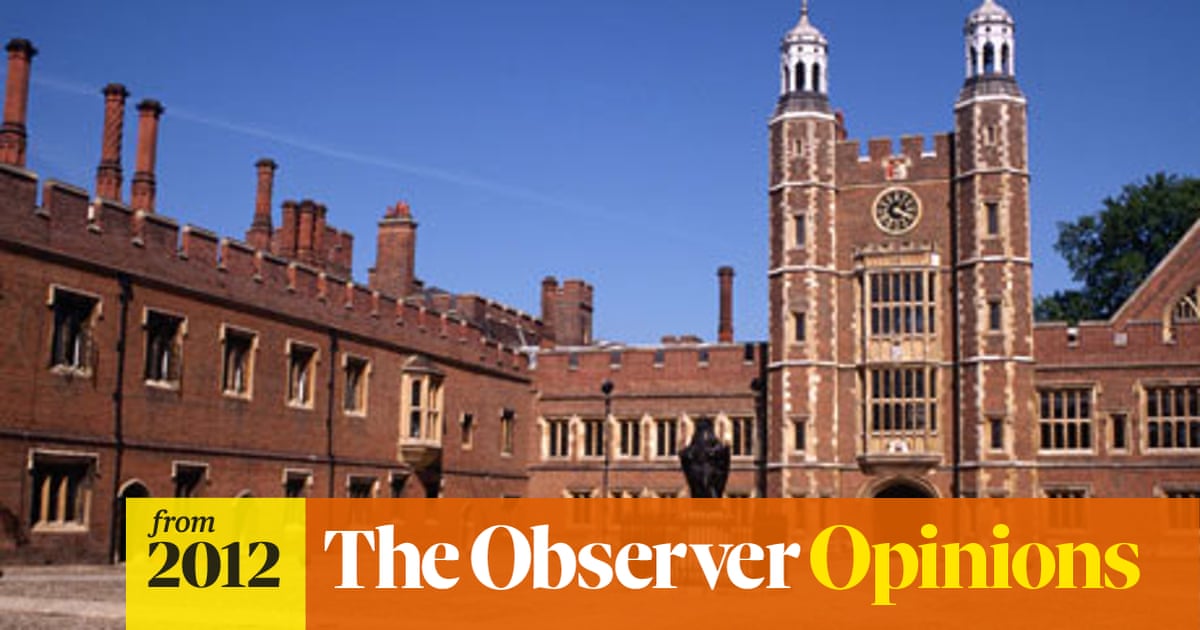This image is a banner for a particular article in The Observer, specifically under the "Opinions" section, as indicated by the text at the bottom that says "From 2012, The Observer Opinions" with "From 2012" in black on a yellow background and "The Observer Opinions" in white on an orange background. The image features an old, majestic red brick building that is likely part of a university campus in England, given the castle-like architectural details, which include a large facade with two prominent towers flanking the primary entrance, each topped with a domed belfry. A notable clock is positioned above the windows, central to the building’s design. The structure is seen against a backdrop of clear blue skies, with a green tree peeking from the right side, enhancing the picturesque outdoor setting.